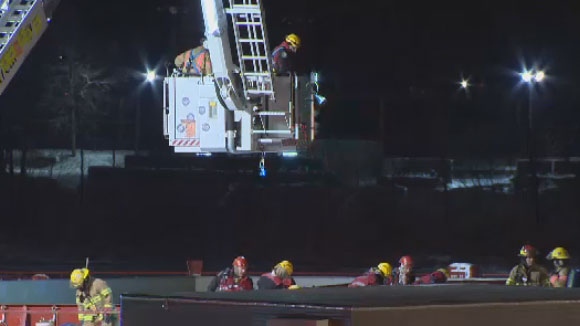A nighttime scene featuring a distant view of streetlights, approximately three to four in number, casting a soft glow over a grassy hillside dotted with trees. In the foreground, a team of rescue workers is diligently operating. Among them, several firefighters are easily identifiable by their yellow helmets and distinctive brown jackets adorned with yellow stripes. Additionally, there are personnel wearing red helmets, contributing to the scene. At the very bottom of the photo, partially obscured, is the top portion of a vehicle, possibly a bus. Dominating the center of the image is a ladder truck, equipped with an elevated lift box. Inside the lift, two figures are visible; one wearing a yellow helmet, while the other’s head is obscured by the machinery. The scene captures a moment of coordinated emergency response, brimming with professional activity against the serene backdrop of a nighttime landscape.